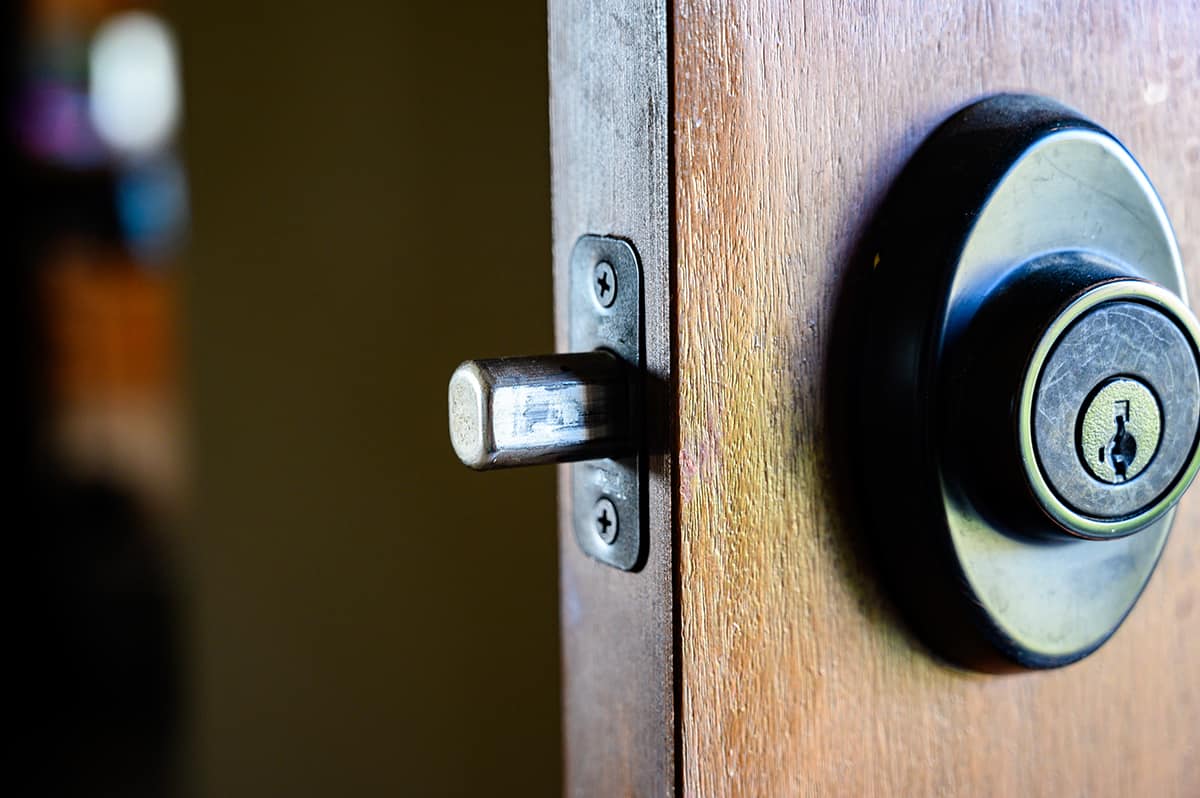This image is a close-up color photograph of a partially open mahogany door stained a rich brown color. The focus of the image is a brushed aluminum deadbolt lock with brass accents, including a brass keyhole which requires the key to be inserted upside down to unlock. The lock features an oblong, raised oval plate with a round brass part inside it, and a metal key slot at the center. The deadbolt is visibly extended from the door, secured by two Phillips-head screws. In the blurry background through the crack of the door, a lit-up room is vaguely discernible, displaying indistinct objects illuminated by direct light.